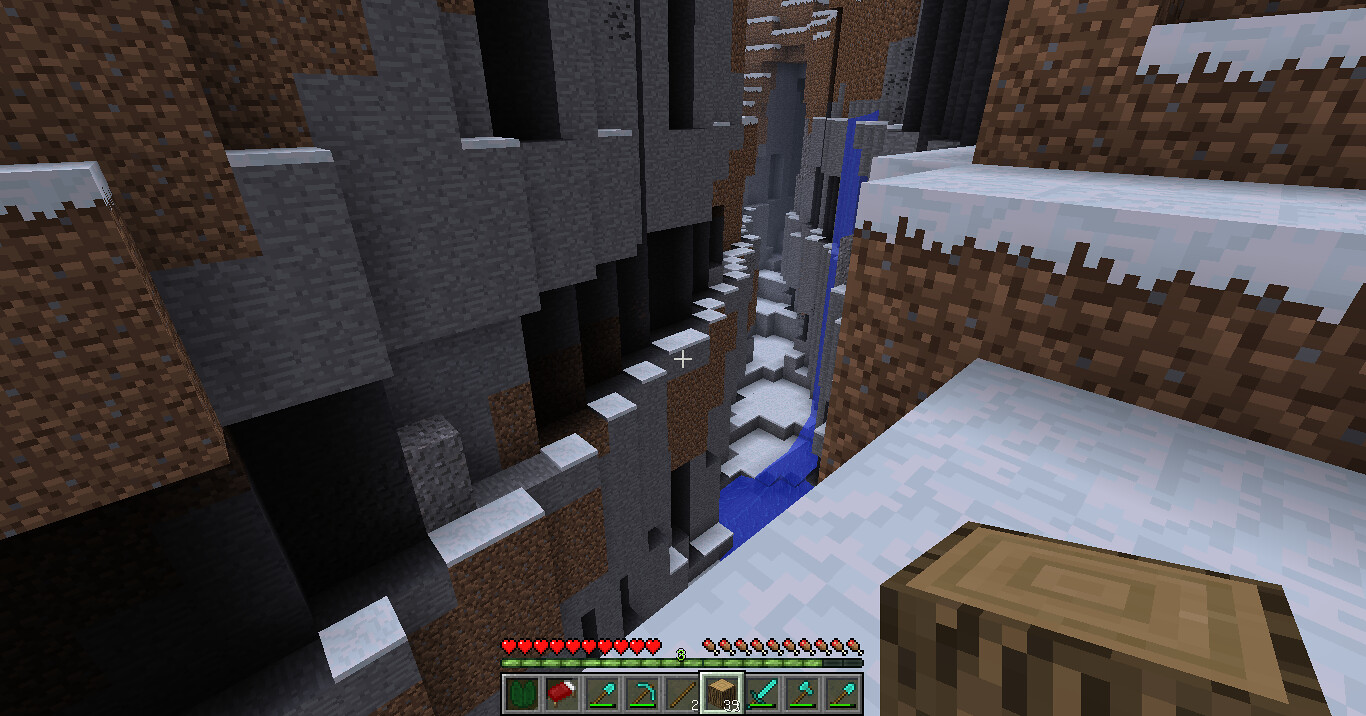The image is a screenshot from the game Minecraft displaying the game's User Interface (UI) and a detailed mountainous landscape. The UI at the bottom center of the screen shows a row of nine inventory slots each containing various items like blocks, swords, and building materials used for crafting. Above the inventory slots, there is a health bar represented by red hearts as well as a food meter depicted as meat sticks with a bone on the end. 

The scene itself is detailed and showcases a tiered landscape with brown rocky steps and ridges, alongside a narrow, cavernous walkway flanked by high walls. Snow covers parts of the ground and the tops of brown and gray blocks, adding a wintry layer to the setting. To the right of the screen, an icy waterfall or stream of water cascades down into the cavern. The viewpoint is from the perspective of the Minecraft character, although the character itself is not visible in the shot.